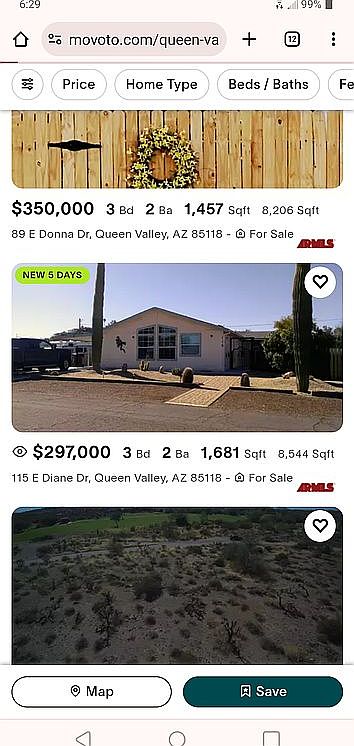Screenshot of a real estate listing webpage on Mavodo.com

The webpage displays a search bar at the top with the URL "mavodo.com/queen-va," accompanied by a small home icon, a "+" symbol, and the number "12" within a square. Below the search bar are various filter options including icons and buttons labeled "Price," "Home Type," "Beds," "Baths," and "FE" (assumed to stand for features).

The first listing features a photograph of a door adorned with a wreath of yellow flowers on a fenced property. Details include:
- Price: $350,000
- Bedrooms: 3
- Bathrooms: 2
- Interior: 1,457 sqft
- Lot: 8,906 sqft
- Address: 89 East Donna Drive, Queen Valley, AZ 85118
- Status: For Sale

This listing also has a "New" tag in green, indicating it was listed five days ago. The accompanying image depicts a small white ranch home with large windows, a spacious road in front, tall shrubs, and a clear blue sky.

The second home listing provides:
- Price: $297,000
- Bedrooms: 3
- Bathrooms: 2
- Interior: 1,681 sqft
- Lot: 8,544 sqft
- Address: 115 East Diane Drive, Queen Valley, AZ 85118
- Status: For Sale

It also features a small, unreadable red logo. Below these listings is an image of a scrubby desert landscape with a road running through it.

Additional page elements include a white "Map" button and a dark green "Save" button. The bottom of the screen presents a navigation bar with triangular, circular, and square shapes on an off-white background.